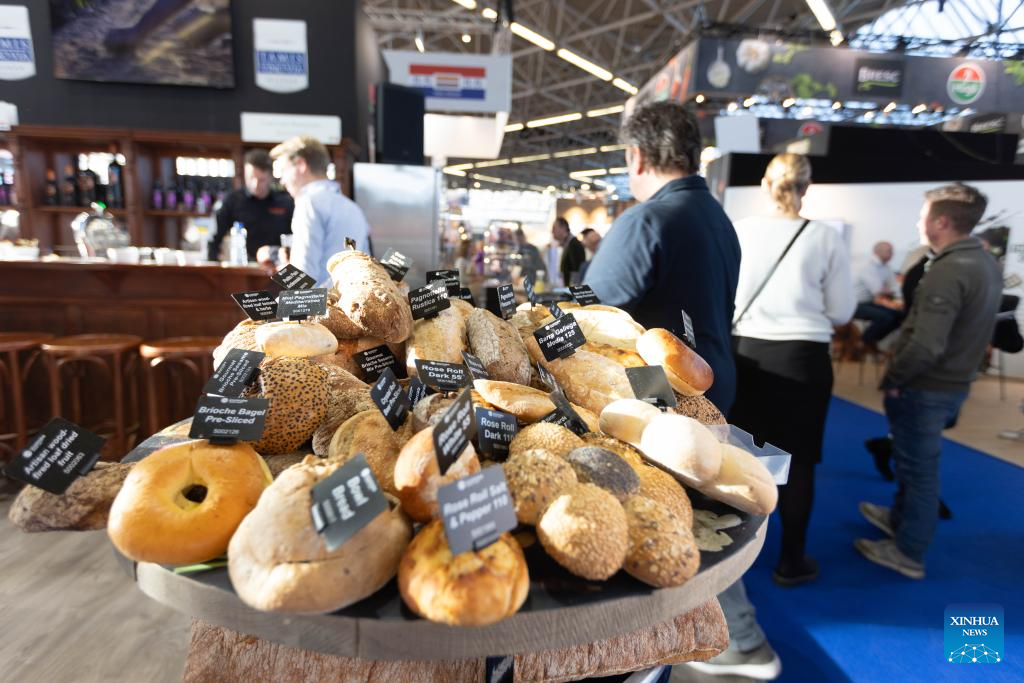The photograph captures an enticing display of assorted pastries, bagels, and buns rolled in seeds, artfully piled on a round serving platter with small signs labeling each variety, though the text is slightly out of focus. The baked goods are set on a weathered wooden table, providing a rustic touch. In the background, the scene is bustling with activity, likely in a convention center or expo with high ceilings and metal rafters. To the left, a wooden bar with stools and visible bottles is attended by an employee, while a customer appears to be placing an order. The setting also includes a business stand with sponsorship logos, where a man seems engaged in a conversation with a client, possibly offering a demonstration. Numerous casually dressed attendees meander around, standing on a bright blue rug that covers the floor. The image, marked with a Xinhua News watermark, vividly captures the dynamic atmosphere of the event.